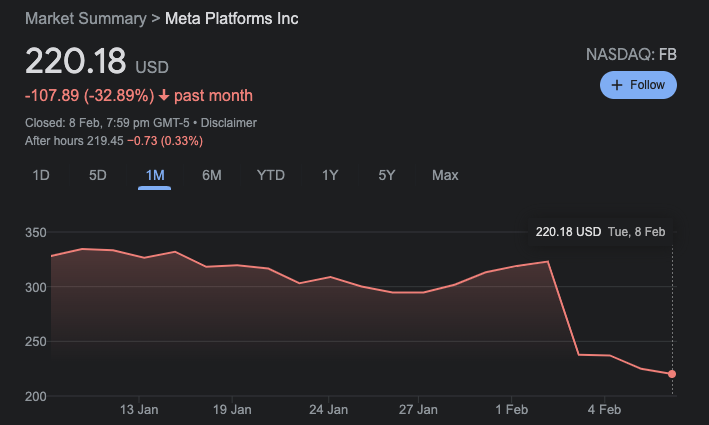Here is the cleaned-up and detailed descriptive caption:

"A screenshot from a financial application or website displaying a market summary of Meta Platforms Inc. (formerly known as Facebook). Set against a sleek black background, the professional interface features 'MARKET SUMMARY' at the top-left corner in grey text. Below it, the company name 'Meta Platforms Inc.' is listed in a slightly lighter grey font, followed by the current stock price of '220.18 USD'. To the right, the information 'Nasdaq: FB' appears, accompanied by a blue 'Follow' button.

The stock performance details indicate a decline, with a value of '-107.89' accompanied by a downward arrow, showing a bearish trend over the past month. The data is valid as of February 8th, with trading details updated until 7:59 PM GMT-5, followed by a standard disclaimer.

The central graph charts the stock performance over various time frames, offering options to view the data for one day, five days, one month, six months, year-to-date, one year, five years, and the maximum duration available. The graph, resembling a typical line or area chart, spans from January 13th to February 4th. The Y-axis scales from 350 to 200, and the line trend indicates that the stock remained fairly steady at around 220.18 USD before experiencing a noticeable drop around February 4th."